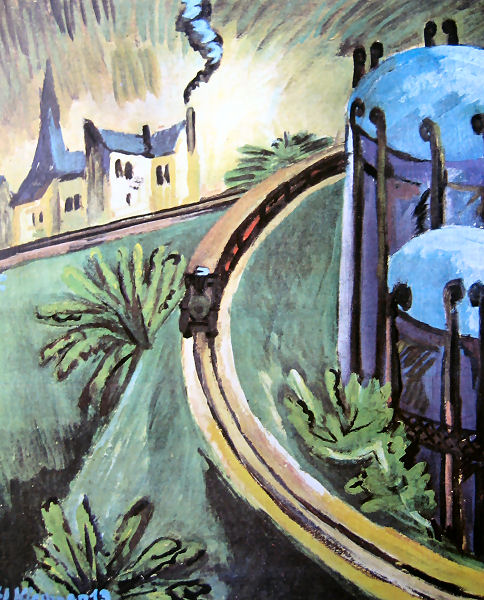This painting, possibly done in watercolors or oil, presents an intricate industrial landscape brimming with detail and color. Dominating the scene is a black, brown, and red train emerging from the right side where it curves around a set of tall, spiraled finial-topped silos colored in blue, purple, and black. The train comes to a halt near the center of the image, continuing to follow a yellow and brown curving track that winds from the bottom right corner. 

On both sides of the track, there's an assortment of greenery – grass with dark shadows and lush green plants, suggesting a possibly tropical setting. To the top left of the composition sits a sprawling yellow house with a black roof, featuring a prominent chimney with gray smoke billowing up from it. This house, possibly a large residential structure or even a church given its size and steeple-like peak, adds to the complex architecture of the scene.

The overall color palette transitions through grays, whites, and yellows at the top, with a striking mixture of greens and earthen hues in the foreground. The painting captures a vivid and almost fantastical industrial environment, detailed with roadways and vivid structural elements that blend into an enchanting and meticulously constructed visual narrative.